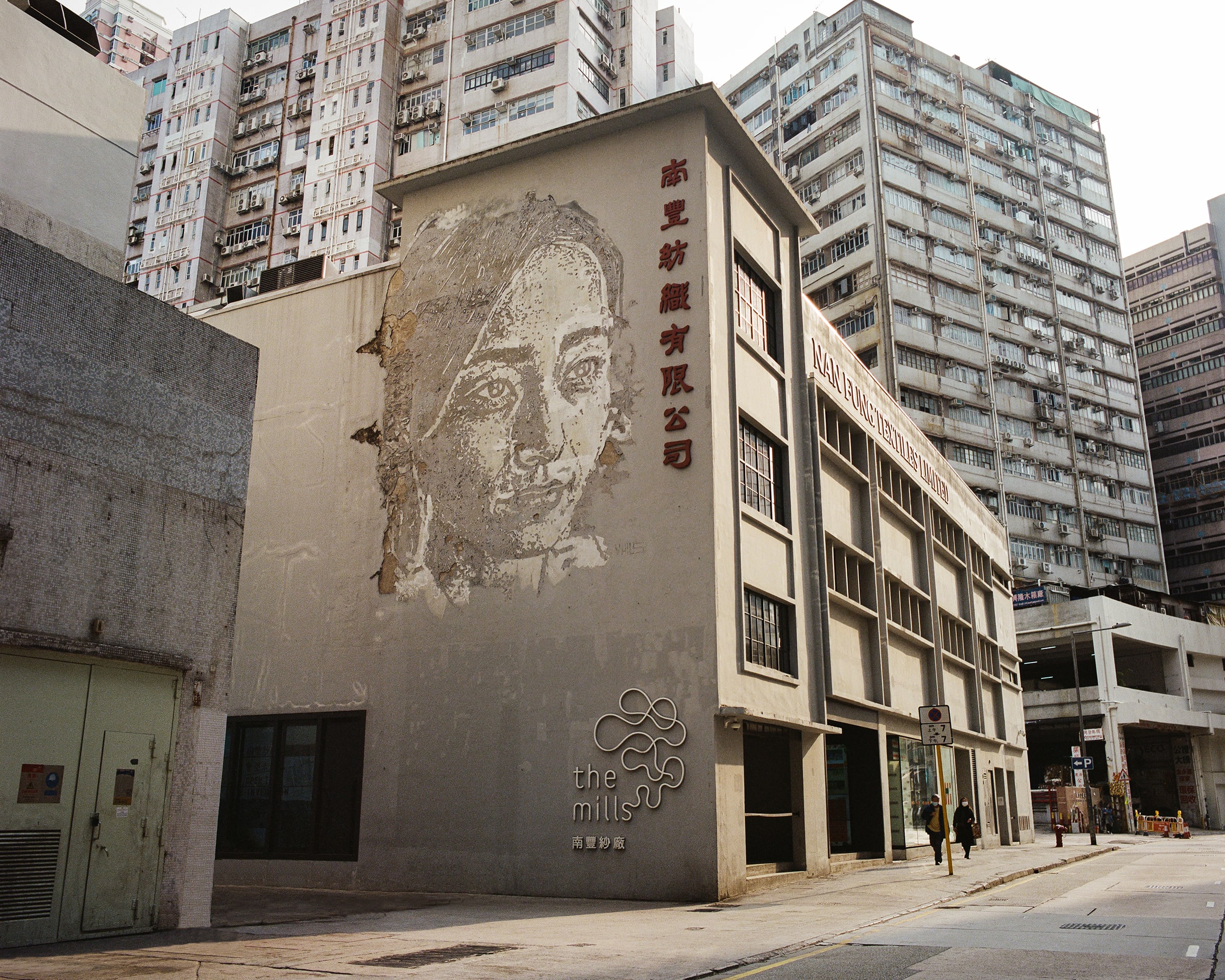The image depicts a dreary city block on a partially sunny day. The central focus is a tan, three-story building featuring a large mural of a young woman with shoulder-length hair and straight eyebrows looking off into the distance. To the right of the mural, several Chinese characters are visible. At the bottom of the mural, the words "The Mills" are displayed, with the trailing 's' extending into a squiggly line containing four additional Chinese characters. To the left of this building stands a very old, dirty stone structure with a green door. Behind and above these structures, an old high-rise building, likely a tenement, is visible, characterized by rows of windows and balconies, with many air conditioners jutting out. Part of a parking structure can also be seen. On the sidewalk in front of the buildings, two indistinct people are walking, but there are no cars visible on the street. This scene, presumably located in China, captures the bleak atmosphere of an urban neighborhood.